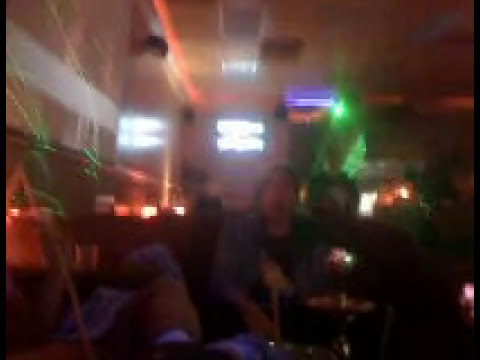In this heavily blurred and out-of-focus photograph, the setting appears to be an indoor space, likely a concert hall, bar, or restaurant. The image depicts a group of people who seem to be standing and socializing, possibly enjoying drinks or taking pictures. Although the exact number of people is uncertain, it is suggested there might be about four individuals. The lighting in the space is varied, with hues of orange, green, blue, white, and red illuminating the scene. Prominent in the background are multiple signs, with white text that is unfortunately unreadable due to the blur. Additionally, there are distinct orange signs positioned both to the left and right of these white statements. An orange flash of light is visible near the top center of the photo, complemented by green splashes of light to the right. In the background, a white wall with some grill work can be discerned. Among the indistinct figures, one person facing the camera appears to be wearing a dark shirt with a coverall and holding an unidentifiable object. To the left foreground, there is a suggestion of a seated individual, with an arm, elbow, and possibly a knee and leg somewhat visible amidst the overall fuzziness.